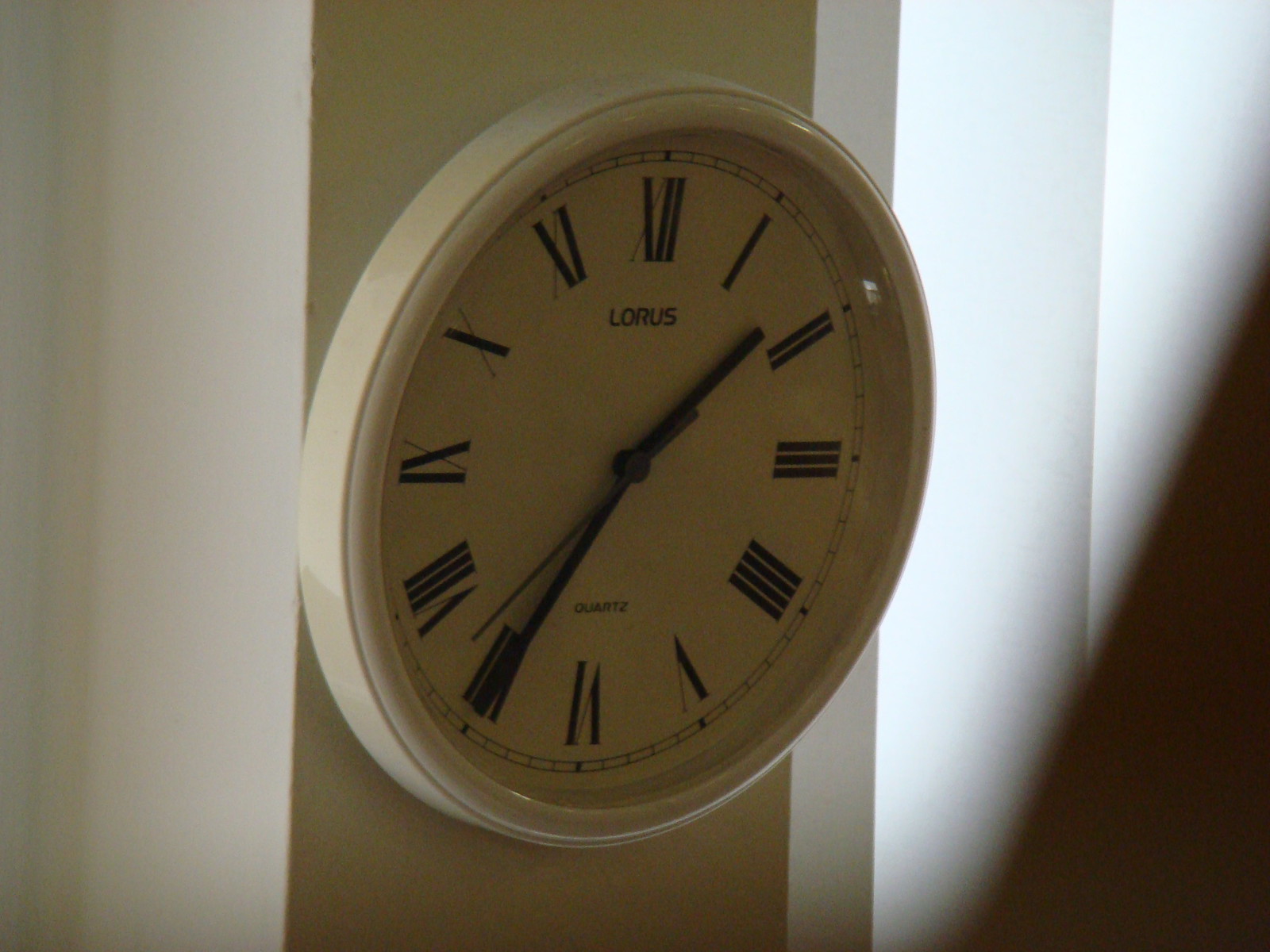This detailed, real-life photograph captures a close-up view of a circular wall clock prominently displayed against a white wall. The clock stands out with its white housing and white face, adorned with black Roman numerals for the hours. The number 12 is represented as "XII," and the number 6 as "VI." Mounted in what seems to be a corner nook, the background includes a white section of wall on the left and vertical blinds that cast lines on the wall to the right. The clock bears the brand name "Lorus" just below the "XII," and "Quartz" is inscribed above the numeral "VI."

The time displayed on the clock indicates approximately 1:35, with the hour hand positioned slightly past the numeral "I" and the minute hand settled on the numeral "VII." The second hand is poised midway between the numerals "VII" and "VIII." Notably, the clock's design is mid-century modern, featuring simple, rectangular black hour and minute hands, and a thin, slightly lighter second hand. The inner frame of the clock face is bordered by two concentric black lines with small vertical notches.

In the bottom-right corner of the image, there's a blurred, up-close object, possibly a finger or another item that obstructs part of the lens, adding a layer of mystery to the image. The photograph has a grainy texture, lending it a vintage feel.